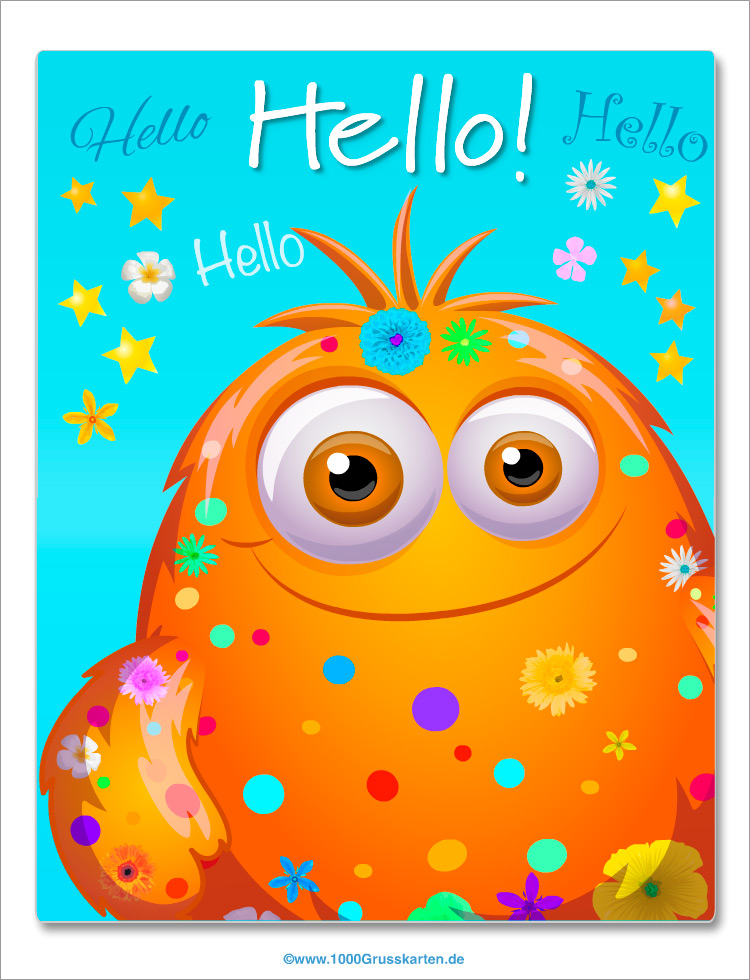The image features an adorable, round, and furry orange monster, exuding a sweet and kind demeanor. Its most distinctive feature is the tuft of hair on its head, styled into five little spikes. The monster’s body is festively adorned with various colored dots and flowers, including patterns in red, yellow, multiple shades of blue, pink, purple, and green. Set against a teal blue background, the scene is further enlivened with scattered yellow stars and colorful flowers. Above the monster’s head, the word "hello" is cheerfully written in four different fonts and styles, suggesting a celebratory or welcoming tone. The overall aesthetic suggests that this could be a greeting card or postcard, with its vibrant colors and lively details, aiming to spread joy and warmth.